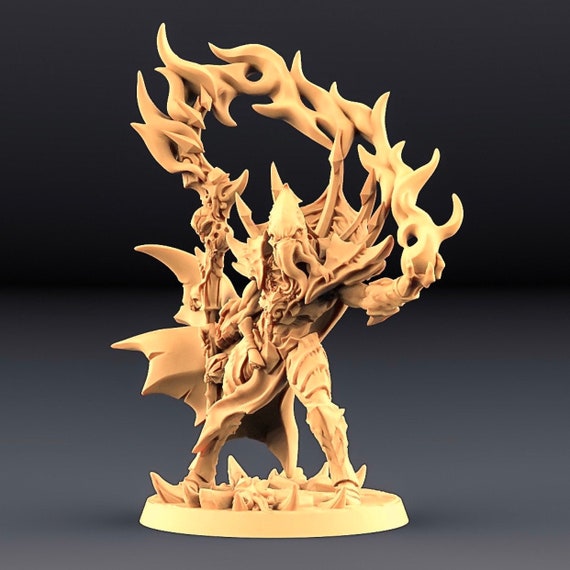In the image, a highly detailed statue, possibly 3D printed, stands against a backdrop that transitions smoothly from black to a very dark gray, adding dramatic emphasis to the figure. The statue, rendered in a consistent tan or bone-like shade, depicts "Slathos the Soul Stealer," a character from Dungeons and Dragons. This creature, structured like a muscular humanoid, has a distinctly non-human face resembling that of a squid.

Slathos, who exudes an aura of mysticism or superpower, is captured in mid-action. He firmly grips a staff in his right hand and raises his left hand to conjure large flames, signifying his formidable magical abilities. He dons an intricately textured outfit with long, sharp, elf-like shoes and pointed ends that enhance his menacing appearance. The entire statue, from the character to the circular stand adorned with simulated rocks and jagged peaks, maintains the same uniform color. Slathos stands poised on this stand, emphasizing his dominance and the supernatural theme of the piece.